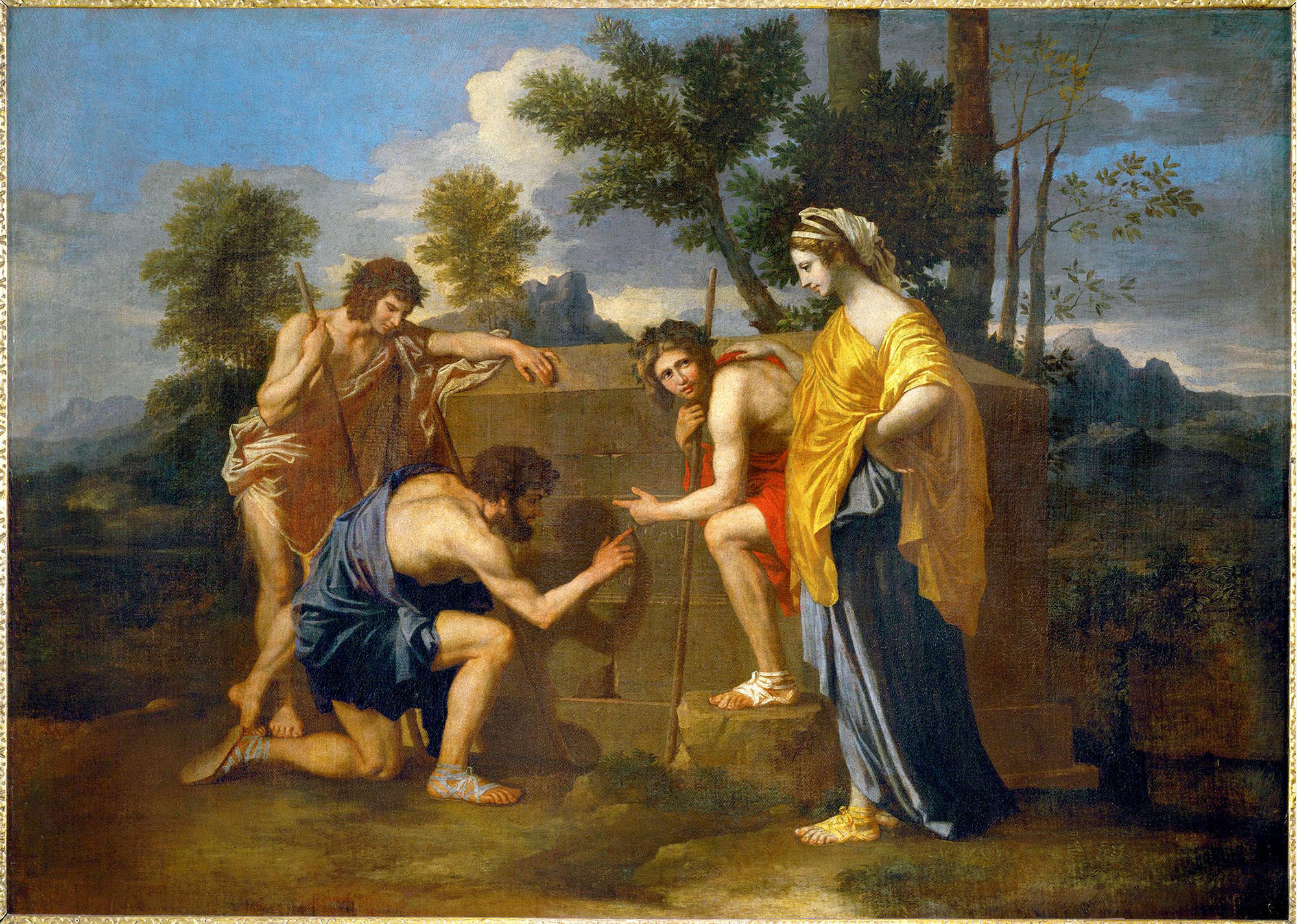This detailed painting, likely from the classical era, features a vivid blue sky punctuated with white clouds and framed by lush green-leafed trees. In the foreground stands a wooden structure, possibly a tomb, surrounded by four figures. The scene includes a man kneeling and using his hand to draw or work on the wooden structure. To the left, a man in a brown cape reveals his chest, arms, and legs, and stands beside another bearded man draped in a blue scarf, his limbs and sandals visible. Further to the right, another man wears a red version of similar attire. The woman, situated on the far right, has dark hair and is adorned in a yellow top paired with a blue skirt, complemented by yellow sandals. She also wears a scarf-like headdress. The painting, characterized by its meticulous detail and classical styling, suggests a scene of significance, potentially interpreted as a biblical moment, and appears to be from the 10th to 16th century.